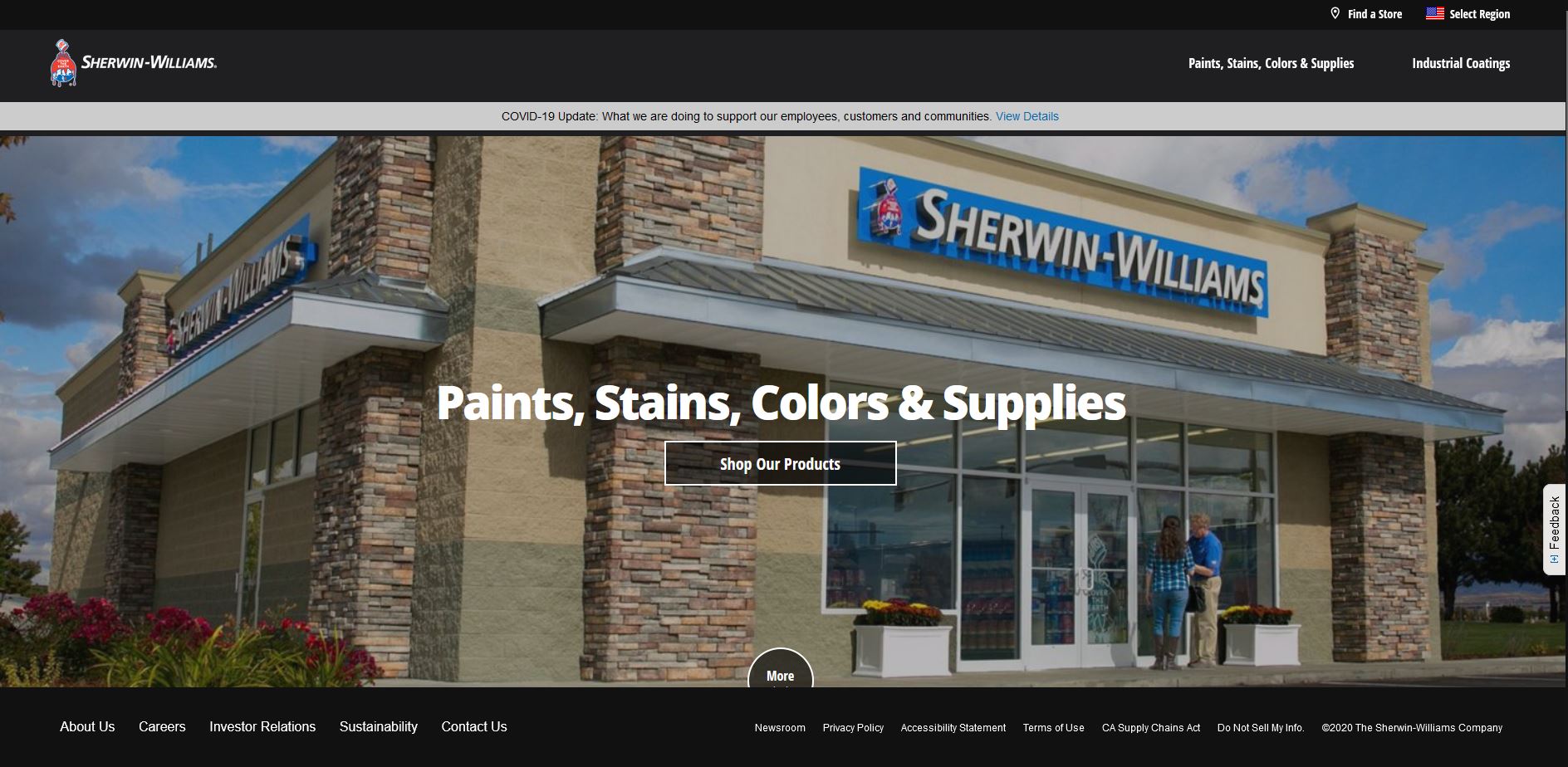This image is a screen capture from the Sherwin-Williams website. At the top, a black banner prominently displays the company's name in white, "Sherwin-Williams," accompanied by its blue and red logo. The navigation bar features links in white to various sections such as "Paints," "Stains," "Colors," "Supplies," and "Industrial Coatings." Above this bar, there is an American flag icon next to the text "Find a Store," marked by a location pin icon.

Below the navigation bar, a gray-and-white banner provides a COVID-19 update in black text: "What we are doing to support our employees, customers, and communities," with a blue link for "View Details."

The central image showcases a Sherwin-Williams physical store. The building is composed of stacked brick columns in shades of brown, tan, gray, and white, with a facade of tan stone. A gray overhang extends from the building. In front of the store, a woman dressed in a blue plaid shirt, jeans, and brown boots, with brown hair, is conversing with a man wearing a blue shirt and tan pants. Two white flower planters containing yellow and burgundy flowers are visible nearby.

In the middle of the image, a text overlay in white reads "Paints, Stains, Colors, and Supplies" within a black box, accompanied by a "Shop Our Products" button and a circular icon labeled "More."

At the bottom, a black banner lists "About Us," "Careers," "Sustainability," "Contact Us," and "Investor Relations" in white text, along with links to the "Privacy Policy" and "Terms of Use." The footer includes a copyright notice dated 2020.